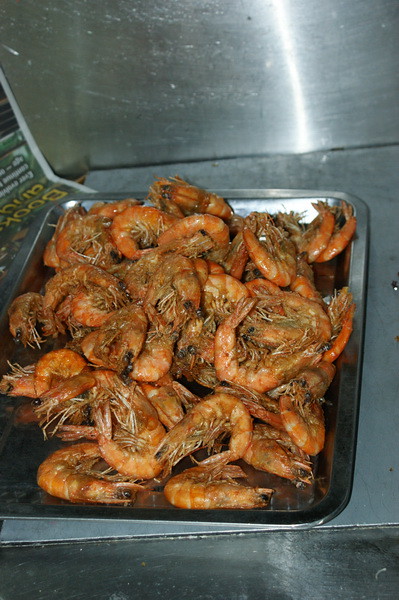This image captures a detailed view likely from a restaurant kitchen. The scene is dominated by metallic, shiny surfaces suggesting an industrial-style cooking area, possibly a grill or prep station. At the center of the photo lies a square, gray tray, gleaming under the kitchen lights. The tray contains a heaping pile of vividly bright orange shrimp, indicating they are fully cooked. Each shrimp retains its shell, legs, heads, and tails. Their signature C-shaped curves are visible, complete with small, round black eyes periodically glinting. In the upper left corner, a green and yellow piece of newsprint or flyer is partially visible, though its contents are indiscernible due to the angle. The overall composition suggests an environment poised for seafood preparation, ready to serve a substantial quantity of shrimp.